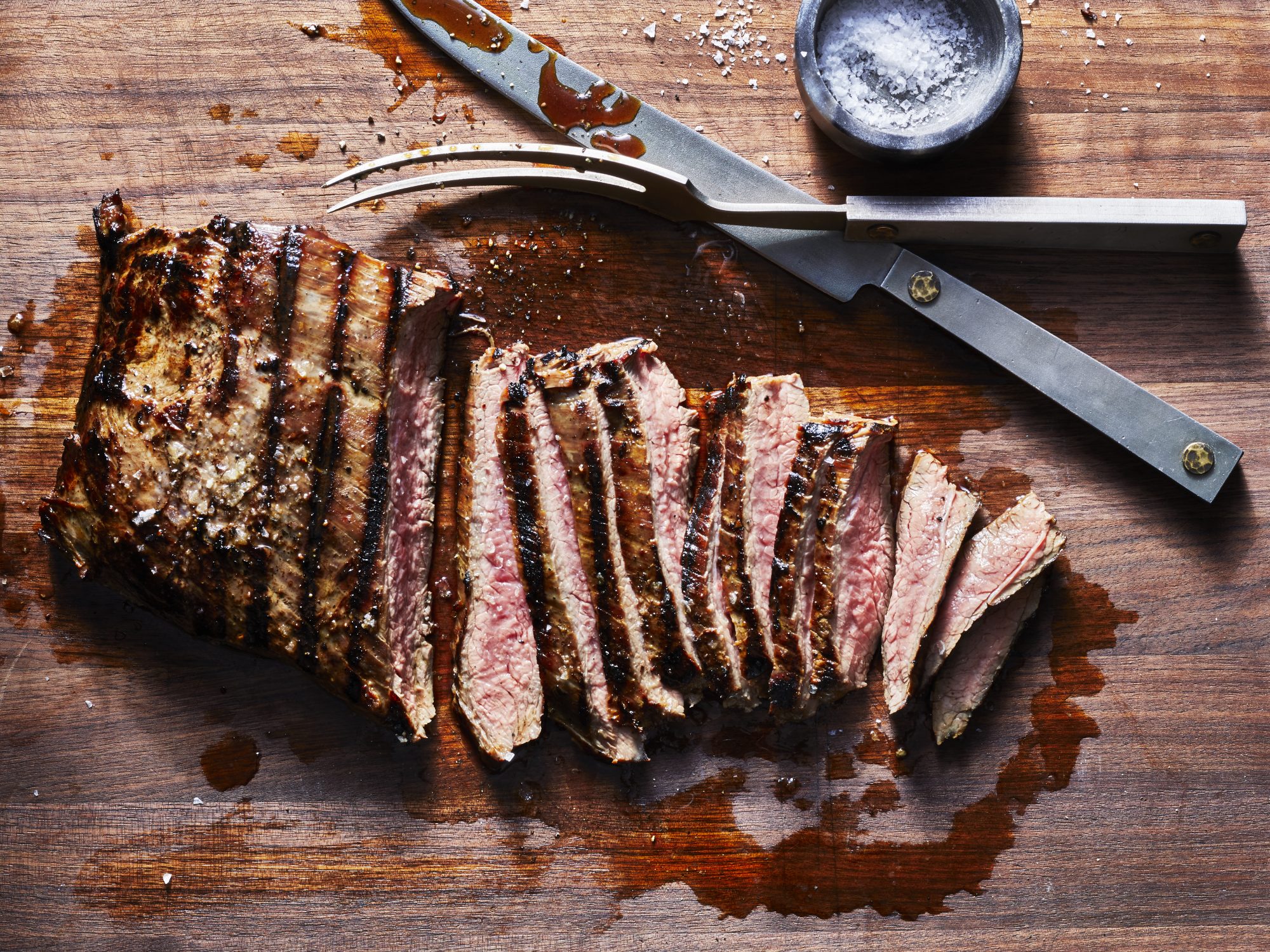This well-lit, overhead color photograph artistically captures a deliciously prepared roast resting on a bright, dry, dark brown cutting board. Occupying the center of the image, the roast has been partially sliced, unveiling a succulent interior with a gradient from pink to brown, suggesting a medium to well-done cook. The roast's exterior is adorned with dark grill marks and glistens under the light, showcasing its enticing texture.

The left side of the roast remains unsliced and is sprinkled with fresh herbs, adding a touch of green and an aromatic hint to the presentation. Juices from the meat have pooled around its base, enhancing the visual appeal with a rich, glossy finish.

A modern metal knife lies flat against the cutting board, its sharp edge smeared with a savory glaze, indicative of careful carving. A matching metal fork rests atop the knife, aligning the silverware diagonally across the bottom right of the roast, further emphasizing the roast's delectable nature.

In the top-right quadrant of the image, a round container filled with either grated cheese or salt adds an extra layer of culinary promise, suggesting forthcoming seasoning. The interplay of light and shadow, combined with the meticulous placement of each element, creates a visually captivating and mouth-watering scene that celebrates the art of cooking.